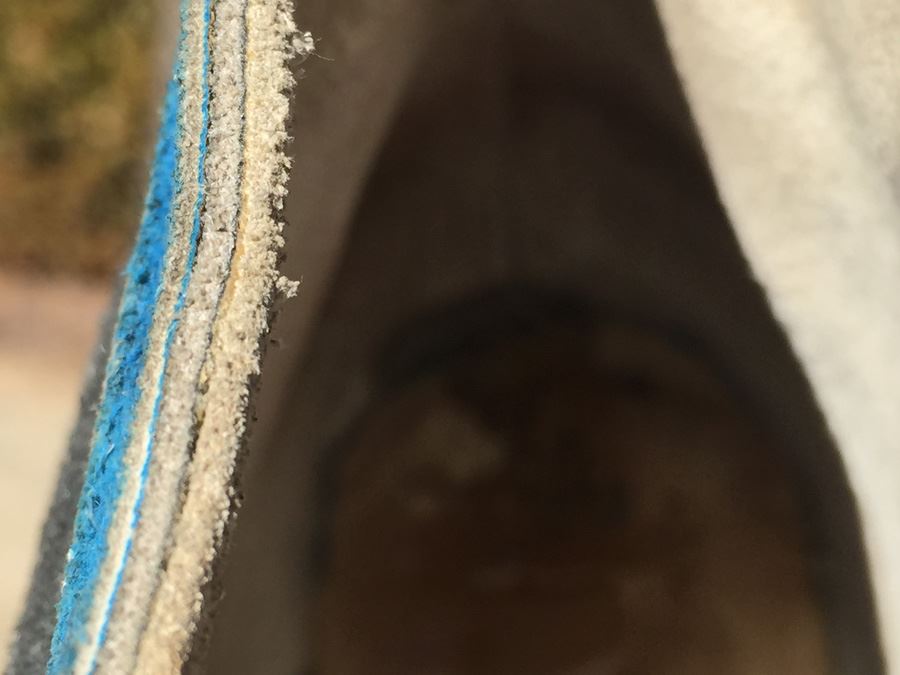This image appears to be a close-up, somewhat abstract view of the inside of a shoe, specifically where the heel is located. The shoe features a distinctive two-tone suede texture, with the right side displaying an almost white suede and the left side a bright turquoise suede. The contrast between these colors is quite stark. The suede sections seem to be meticulously constructed, possibly either glued or stitched together, as indicated by the visible layers and seams. 

The inner bottom part of the shoe shows signs of wear and appears to be made of leather, extending a seam from the bottom to the top at the back. This area is shrouded in shadow, creating a focal dark and somewhat brownish area that deepens in the center, enhancing the abstract quality. A sliver of the fuzzy background, with indistinct shapes in medium tones, can be seen on the left edge of the image. Additionally, there’s a visually distinct, spongy material on the left side, presenting a mix of blues and beige in a vertically layered direction, further adding to the complexity of the composition.